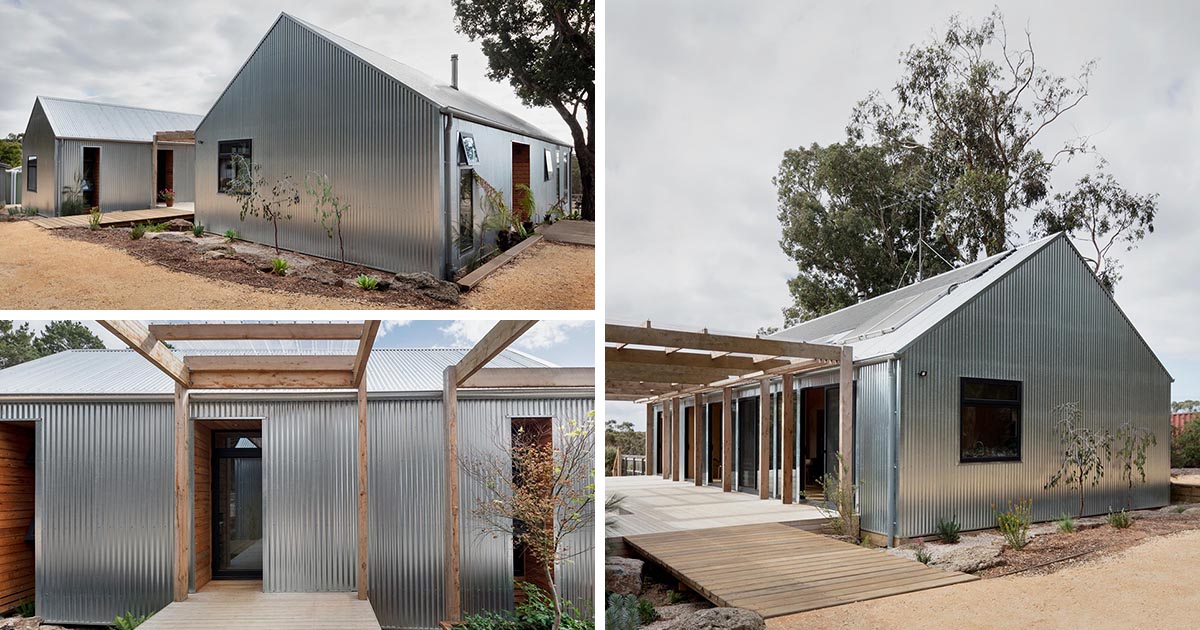The set comprises three photographs showcasing a series of unusual, likely newly built metal buildings situated in a flatland or desert-like area with a sandy, light brown terrain. These structures, gleaming with shiny, corrugated metal on both their roofs and walls, resemble small houses and appear interconnected by wooden decking, possibly forming a small community. The images reveal a construction phase, with ongoing work on a wooden trellis framework, potentially for an additional building. The buildings feature black inset windows and entry doors, with one photograph illustrating open doorways and windows. The surrounding area includes some recently planted greenery, such as small plants and trees, adding a splash of green against the predominantly silver and brown landscape. Tall trees are also visible in the background under a cloudy, gray sky.